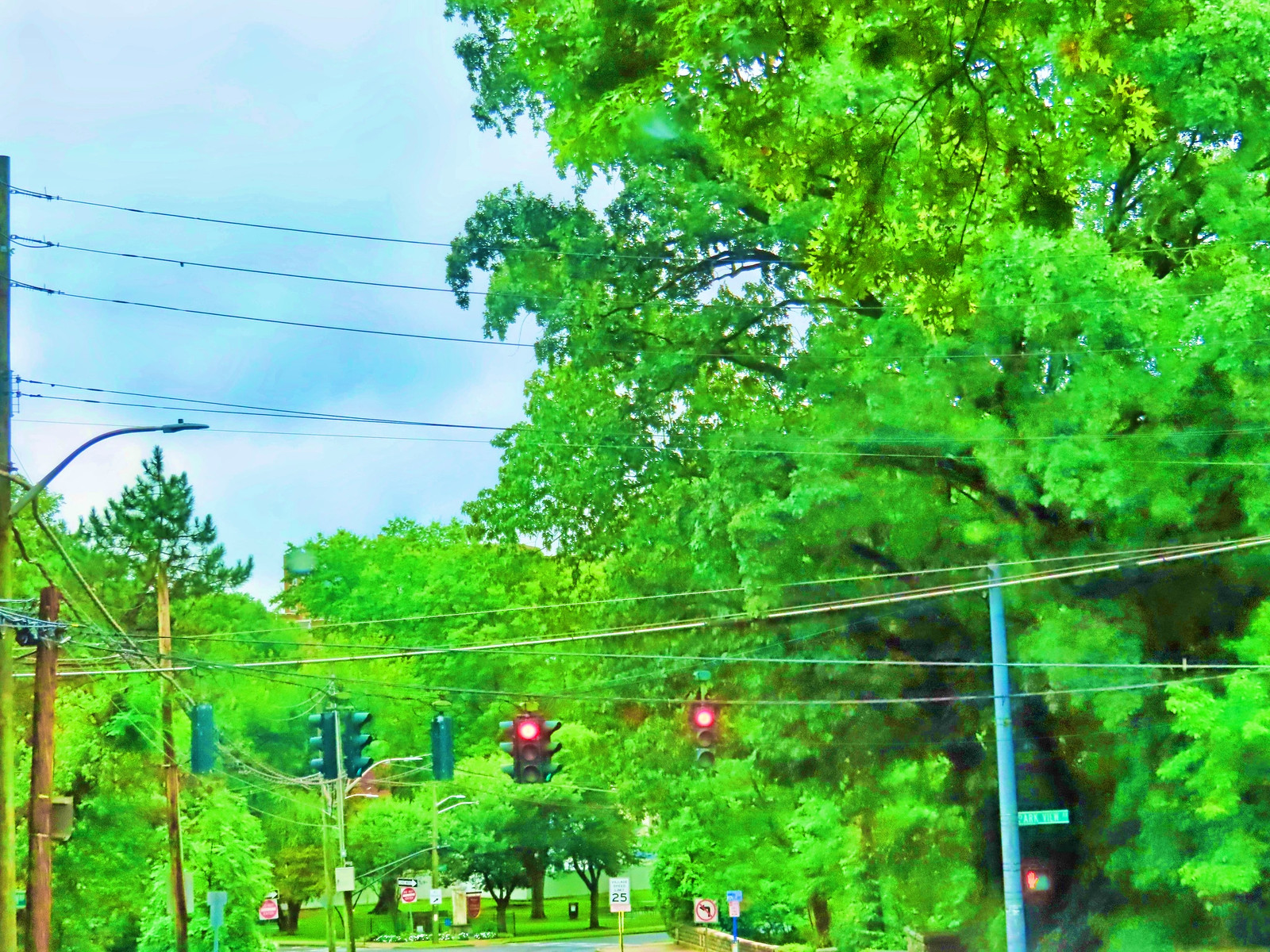The photograph, rectangular in shape with longer top and bottom sides, captures an intricate scene of urban infrastructure. At the bottom of the image, a series of traffic lights dangle from a thin black wire that stretches horizontally from left to right. These traffic signals face multiple directions, although those facing forward currently display red lights at the top, with yellow and green lights below those remaining off. 

Attached to one of the supporting wires is a long metal pole. Midway down the pole, a rectangular green street sign reads "Fair View" in bold white lettering. Further down this same pole is a square pedestrian traffic light, currently illuminated with a red LED figure indicating 'stop.'

To the left side of the frame, a collection of wooden telephone poles stands with an array of black wires extending in multiple directions, adding a chaotic yet structured element to the urban tableau. The composition of the photograph effectively captures the essence of city life with its complex network of functional elements designed to manage both vehicular and pedestrian traffic.